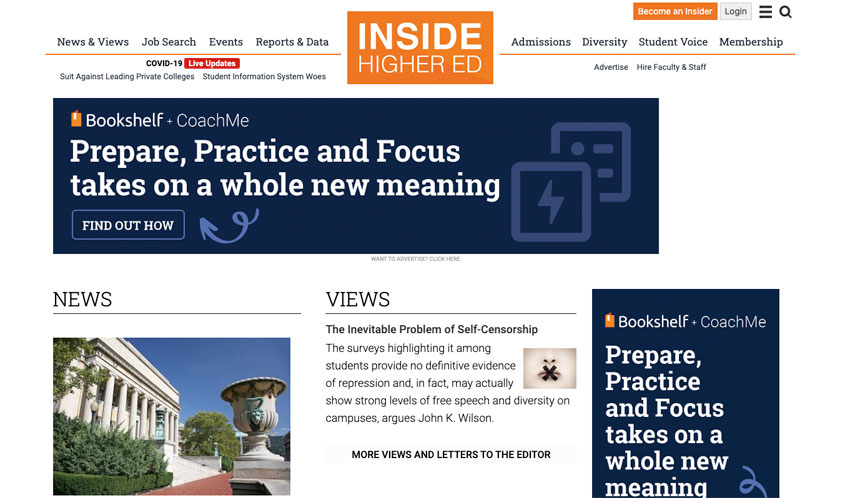This screenshot showcases the homepage of Insider Higher Ed, a website focused on providing news and information related to higher education. The site’s logo, featuring white text within an orange box, is prominently displayed in the top center of the page. 

In the top right corner, several utility buttons and options are available: an orange “Become an Insider” button, a gray "Login" button, a three-line dash icon signifying a menu, and a search magnifying glass icon.

Below these, a horizontal navigation bar allows users to access various sections of the website including: News & Videos, Job Search, Events, Reports & Data, Admissions, Diversity, Student Voice, and Membership.

Further down the page, there is a highlighted section dedicated to COVID-19 updates. This section also includes smaller text mentioning “Suit against leaving private colleges” and “Student information system woes.”

On the right sidebar, advertisements promote the hiring of faculty and staff, with a notably dark blue banner at the bottom labeled "Bookshelf and Coach Me," featuring the tagline “Prepare, practice, and focus. It takes on a whole new meaning.”

The main content area of the page is divided into two columns. The left column, labeled "News," features an image below its heading. The right column, marked "Views," provides the title and introduction to an article discussing the issue of self-censorship.

At the very bottom of the right column, another dark blue rectangular section repeats the "Bookshelf plus Coach Me" ad in a smaller, vertical format.